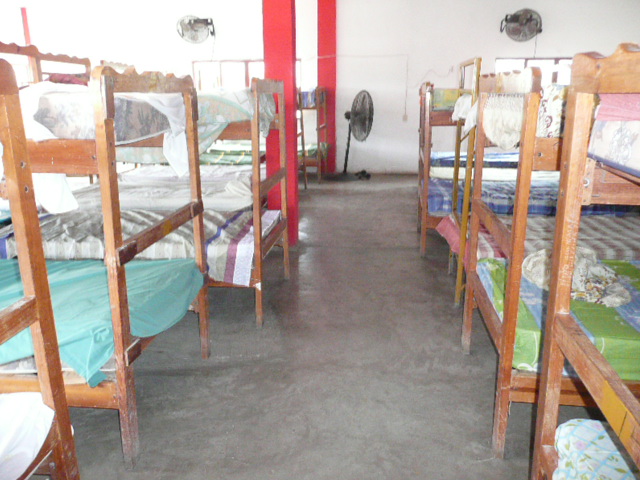The image shows a large room with a concrete floor and multiple wooden bunk beds arranged in two rows with a small aisle in between. The bunk beds have a slightly dusty appearance and each one is equipped with colorful mattress covers. At the far end of the room, a large pedestal fan stands on the floor, suggesting the area might be hot. Additionally, two other gray fans are mounted on the walls at the top left and top right corners of the image. The far wall is white, and there are red pillars descending from the ceiling throughout the room. This setting, with its mix of colorful bedding and multiple cooling fans, hints at a communal sleeping area possibly used for a summer camp or a facility caring for children.